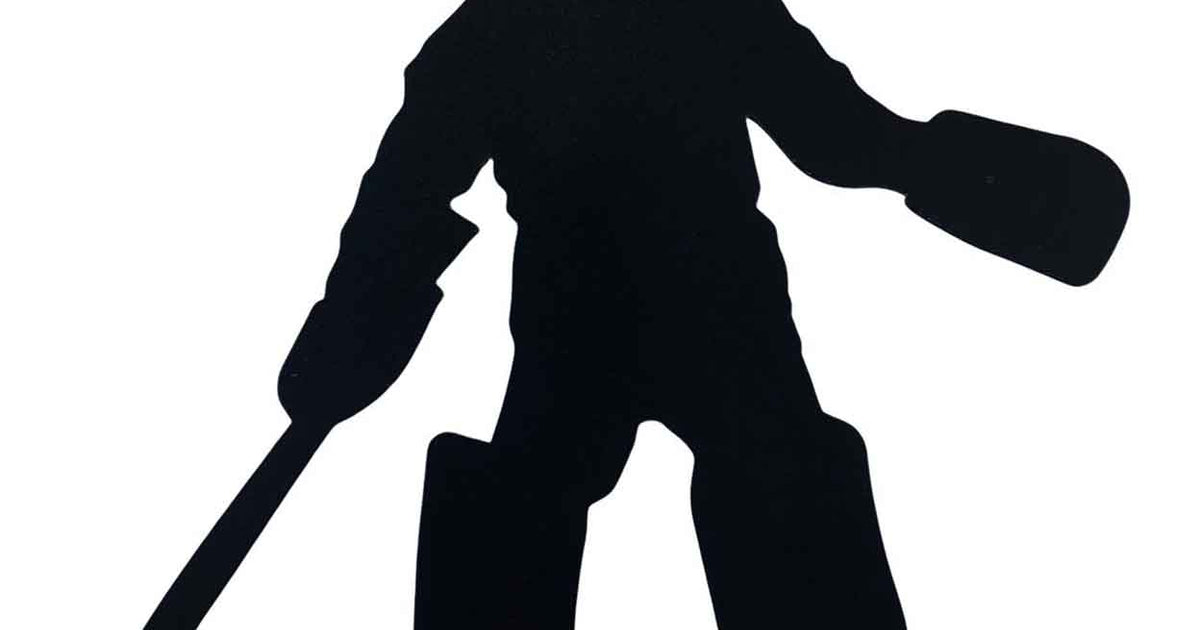The image displays a striking silhouette of a character that closely resembles a hockey player clad in full uniform. This black silhouette against a stark white background creates a high-contrast, minimalistic aesthetic. The image is cut off at the shoulders and just above the knees, leaving the head and feet obscured. The character's left hand is slightly raised, while the right hand is bent down and holds what appears to be a stick or similar object, suggestive of a hockey stick or possibly even a sword. The left hand seems to be adorned with a mitt, and although the feet are not visible, there are protrusions at the bottom of the legs that give the impression of boots. The overall composition is simple yet evocative, with no additional text or colors to distract from the stark, graphic outline of the silhouette.